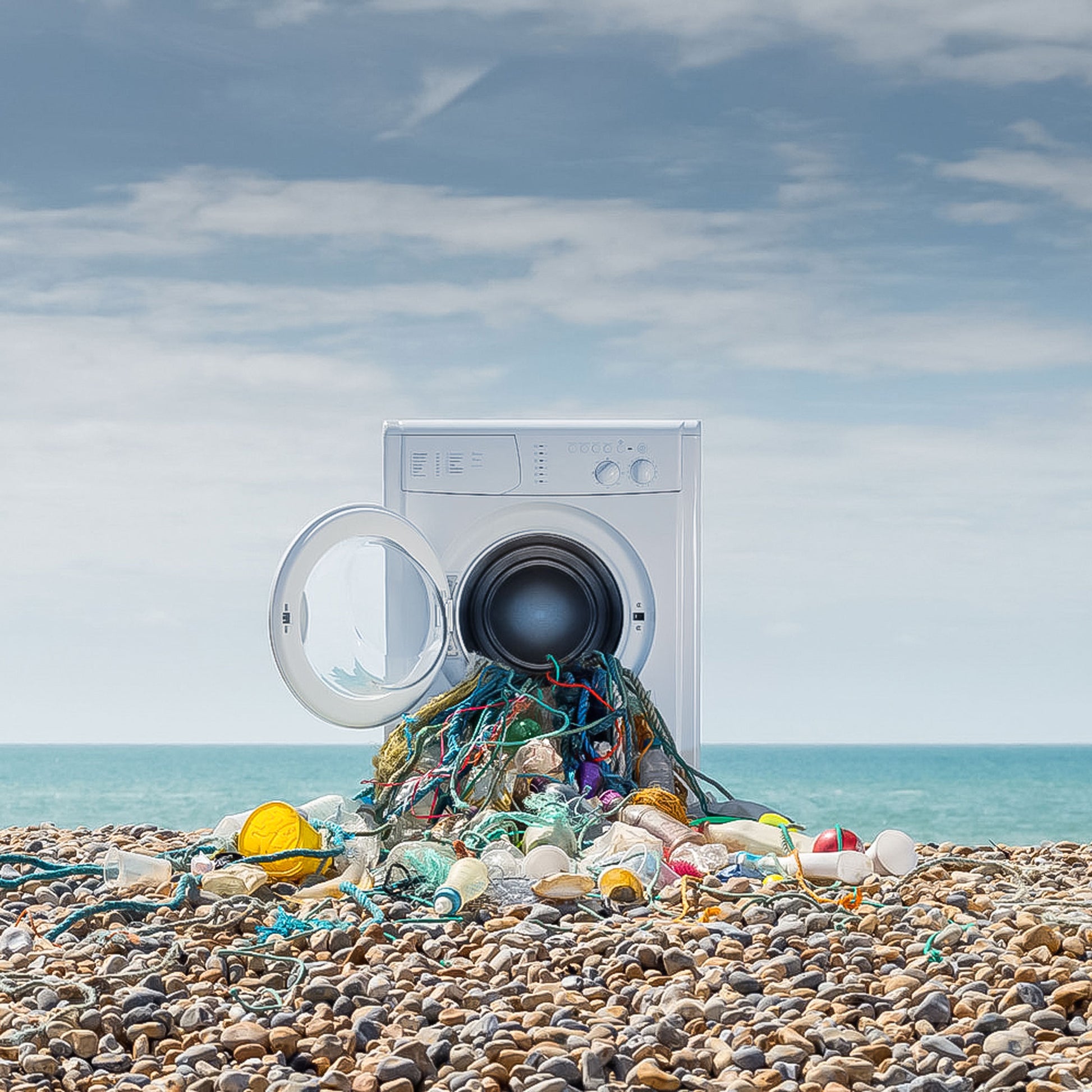In this detailed visual illustration, a white front-loading washing machine is depicted sitting on a rocky, pebble-strewn beach near the ocean. The washing machine's door, which has white knobs and transparent glass, is wide open, revealing a jumbled mass of waste materials spilling out onto the shoreline. The debris includes various colored ropes, fishing nets, plastic bottles, clear and white cups, and other plastic trash such as yellow buckets and red items. The background showcases a serene, light blue ocean under a partly cloudy sky, with feathery white clouds scattered above. The gray and tan rocks on the beach highlight the stark contrast between the clean ocean scenery and the pollution emanating from the washing machine. This powerful image likely computer-generated, emphasizes the pressing issue of ocean pollution.